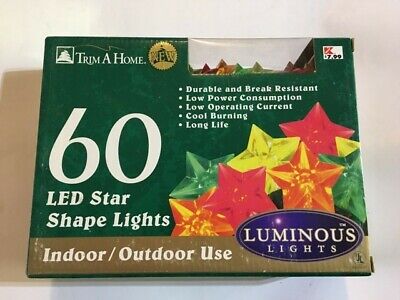The photograph depicts a low-resolution, low-quality image of a green, cardboard box of Christmas lights positioned on a white surface. The top left corner of the box features the brand name "Trim-A-Home" with a prominent gold "NEW" stamp. A clear cellophane window on the front allows a glimpse of the star-shaped LED lights inside, which come in orange, green, red, and yellow. The box also has an illustration of the lights, emphasizing their five-pointed star shape. Priced at $7.99, as indicated by a Kmart sticker, these lights boast features such as durability, break-resistance, low power consumption, low operating current, cool burning, and long life. The packaging highlights that there are 60 LED lights, suitable for both indoor and outdoor use, and they are branded under "Luminous Lights" within a purple circle on the box.